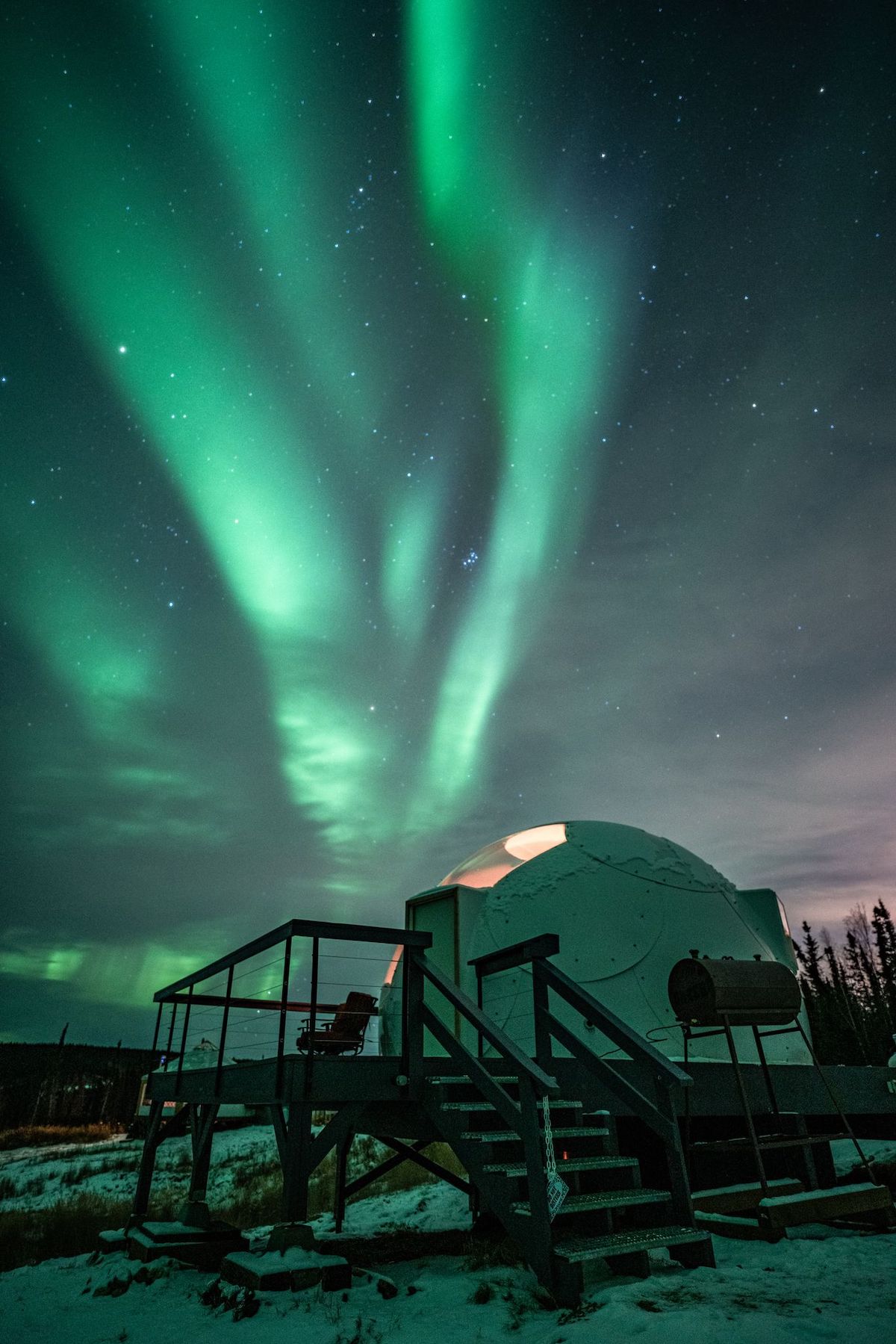The photograph features a dome-shaped observatory with a wooden deck and a chair outside, set against the mesmerizing backdrop of the Aurora Borealis. The structure, colored white and beige with overlapping sheets of circular metal, is elevated above a snowy ground, suggesting a winter setting. The sky is dominated by a stunning light phthalo green aurora that streaks across and through the sky, creating a misty haze. Accents of cyan and occasional pinkish blue hues mix with the green, adding depth and variation to the celestial display. The dark sky behind the aurora transitions from light to dark, punctuated by variously sized and bright stars represented as little white dots. On the right side of the image, a line of trees borders the scene, and another building, dark brown or black, appears to the left, with a portion of the aurora filtering above it. Warm, glowing light emanates from the observatory’s interior, adding a cozy touch to the otherwise icy and serene landscape.